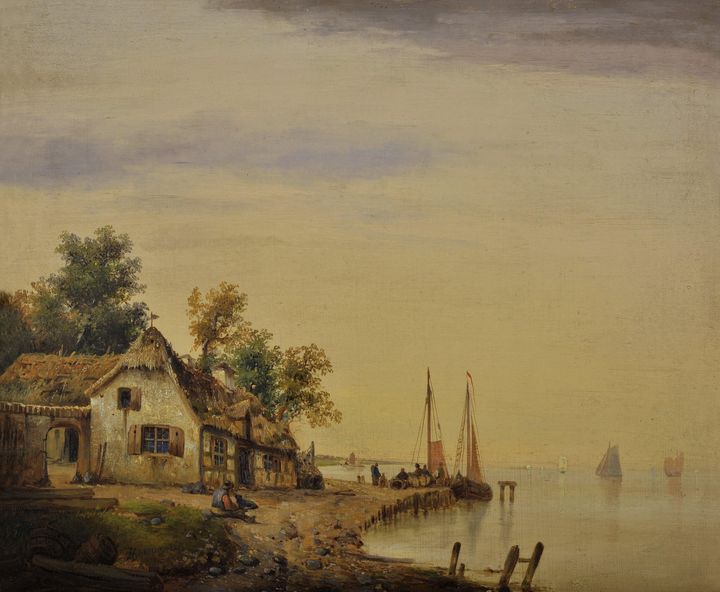This painting depicts a serene sea-to-shore scene featuring a quaint, off-white house with a thatched roof and brick walls, positioned right at the edge of a wooden pier. The house has two windows and a door at the front facing the water, with an additional window with shutters on the side. An archway on the left side leads through a cement wall into a backyard area where brooms or debris can be seen. 

In the immediate foreground, a man wearing a red shirt and blue vest is seated on the ground with his legs stretched out on the dirt, possibly with an animal beside him. There is some grass behind him with scattered wooden logs. Behind the house, lush green and yellow-leaved trees are visible.

The water is animated with several sailboats: two with red and white sails docked near the pier, and others with blue, red, and white sails further out on the slightly choppy waters of the sea or lake. The upper part of the scene is dominated by a mostly cloudy sky with only minor patches of blue peeking through and darker clouds suggesting an impending twilight. This idyllic view is reminiscent of an old seafaring village, capturing the tranquil yet bustling life by the shoreline.